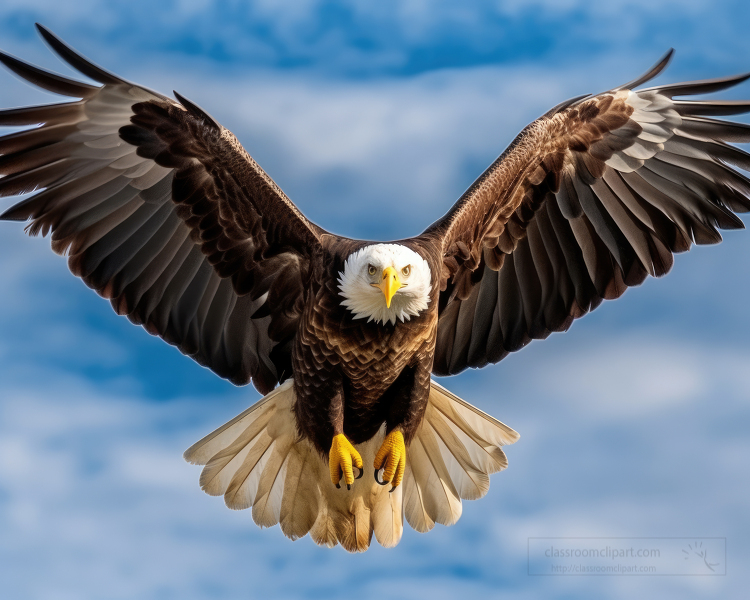In this striking image, a magnificent bald eagle dominates the frame, captured mid-flight with its massive, dark brown wings fully outstretched. The contrasting white head and sharp, angled yellow beak, adapted for breaking bones, are prominently visible. The eagle's piercing eyes are focused away, likely on its prey, as its powerful, bright yellow talons, tipped with formidable black claws, are ready for the hunt. The eagle's body shares the same rich brown tones interspersed with lighter brown and white feather detailing. The background reveals a cloudy sky, blending bluish and whitish hues, suggesting a typical midday setting with ample daylight.